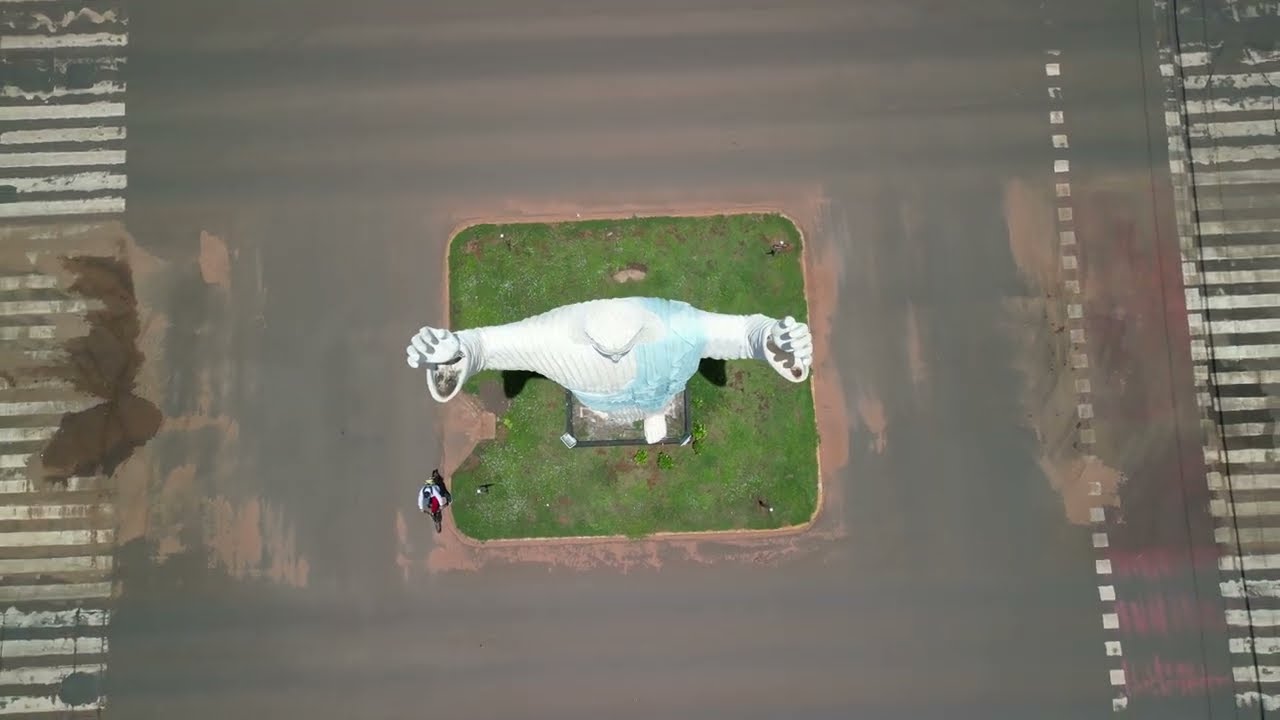This is a detailed, aerial daytime photograph showing the iconic white Christ the Redeemer statue in Rio de Janeiro, Brazil, captured in a landscape orientation. The image, taken from a drone, looks directly down at the statue, which stands at the center with its arms outstretched over a square patch of green grass. Surrounding the grass is a broad expanse of gray pavement, possibly a road or parking lot, marked with white stripes on both the left and right sides. At the bottom left corner of the grassy area, a man is visible, walking away from the viewer. The overall style of the photograph is realistic and representational, emphasizing the artistic and meticulous geometric composition of the scene. The colors in the image include shades of white, gray, green, light blue, and tan.